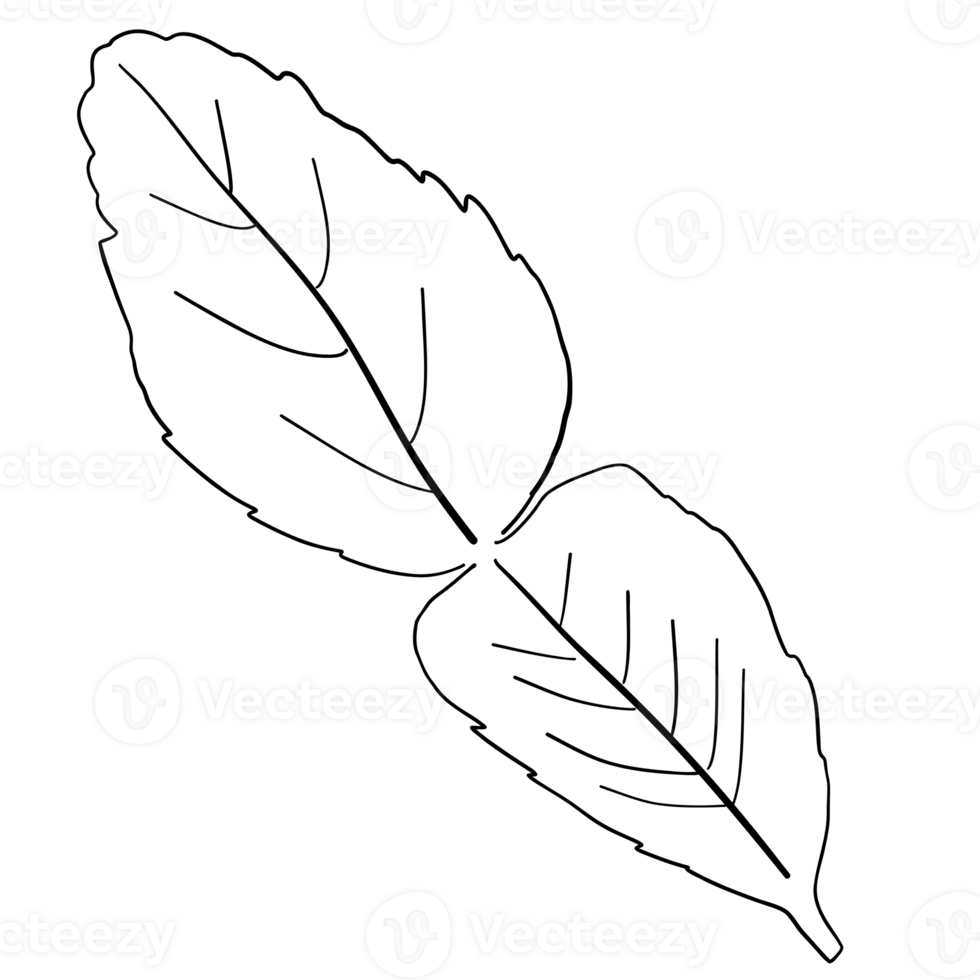The image presents a very simple black-and-white line drawing of two leaves against a stark white background. This childlike sketch is characterized by its rudimentary, yet unmistakable, representation of the leaves, each outlined distinctly. The leaves are connected, with one overlapping the other in an almost V-shaped formation. The central vein of each leaf is prominent, depicted with a thicker black line, while thinner lines branch off to mimic the natural vein patterns. The bottom leaf features a central vein with five smaller veins extending upward and three downward, while the top leaf showcases three veins on either side of its central line. The edges of the leaves appear slightly broken and ragged, adding to their simple charm. Above the drawing, there are faint watermarks from Vecteezy, a stock image site, including the name "Vecteezy" and a logo featuring a squiggly V inside a circle, both subtly repeating across the image.